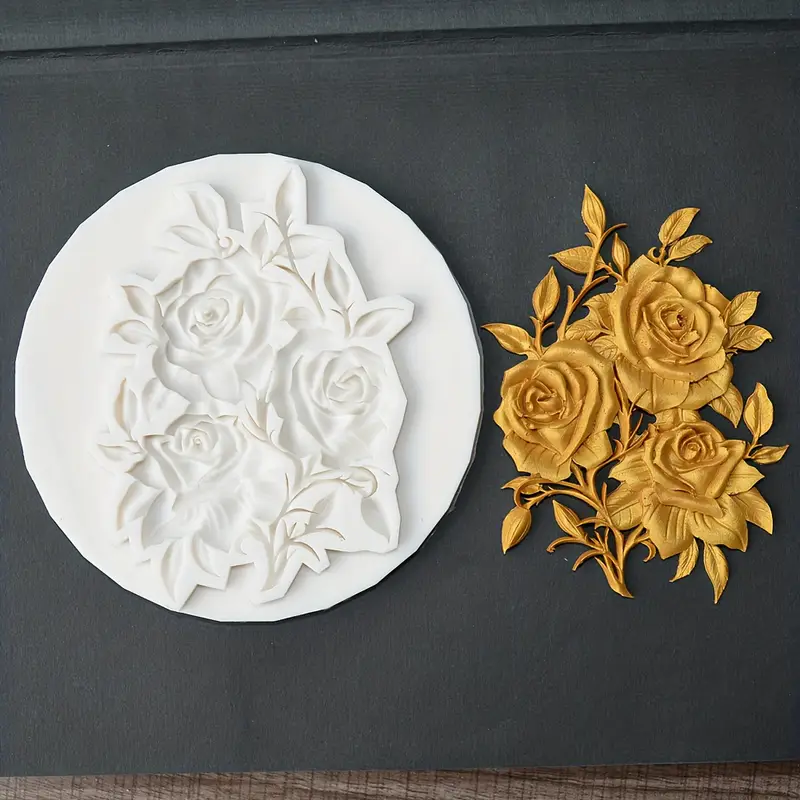A detailed photograph showcases a charcoal gray background displaying two intricately designed carvings. On the left side, there is a large, circular white plaster mold featuring a deeply etched and raised bouquet of three roses, made visible through delicate gray shading. The intricate design within the mold includes detailed petals and leaves suggesting an embossed bouquet. To the right, placed on the same background, is the final product cast from the mold, a cluster of three roses with short stems and leaves, carved in a golden, tannish material. The realism of the golden bouquet highlights the detailed craftsmanship possible with the mold. The overall setup is enhanced by a very thin, dark brown wood grain banner at the bottom of the frame, adding a subtle touch to the presentation.